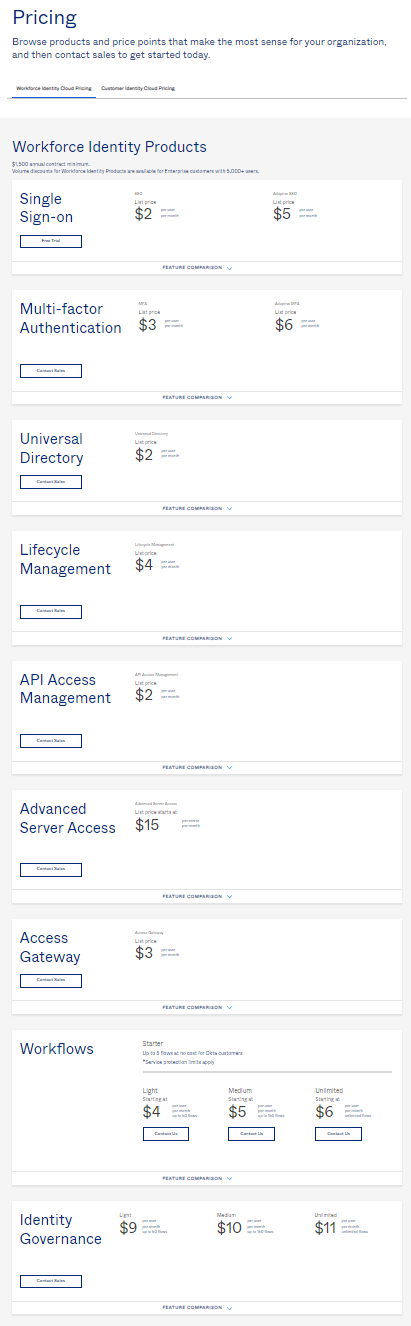This image captures a detailed pricing table from a technical product website, displayed predominantly in black and blue text on a white background. At the top of the table, the heading in blue reads "Pricing," followed by a subheading encouraging users to "Browse products and price points that make the most sense for your organization" and to "contact sales to get started today."

The table is divided into several sections, with each section listing various workforce identity products and associated pricing tiers. The "Workforce Identity Products" section is detailed as follows:

- **Single Sign-On:** $2 for the basic tier and $5 for the advanced tier.
- **Multifactor Authentication:** $3 for the basic tier and $6 for the advanced tier.
- **Universal Directory:** $2.
- **Lifecycle Management:** $4.
- **API Access Management:** $2.
- **Advanced Server Access:** $15.
- **Access Gateway:** $3.

In addition, there are workflow options:
- **Workflows:** Light at $4, Medium at $5, and Unlimited at $6.
- **Identity Governance:** Light at $9, Medium at $10, and another tier priced at $11.

Beneath each of these product listings are columns of checkboxes likely intended for feature comparison, although the text within these checkboxes is too small to read even at a high zoom level.

Despite the difficulty in reading some smaller text elements, the table evidently serves as a comprehensive guide for potential customers to understand various product options and select services tailored to their organizational needs. This screenshot appears to be a segment from a tech product or identity management service website.